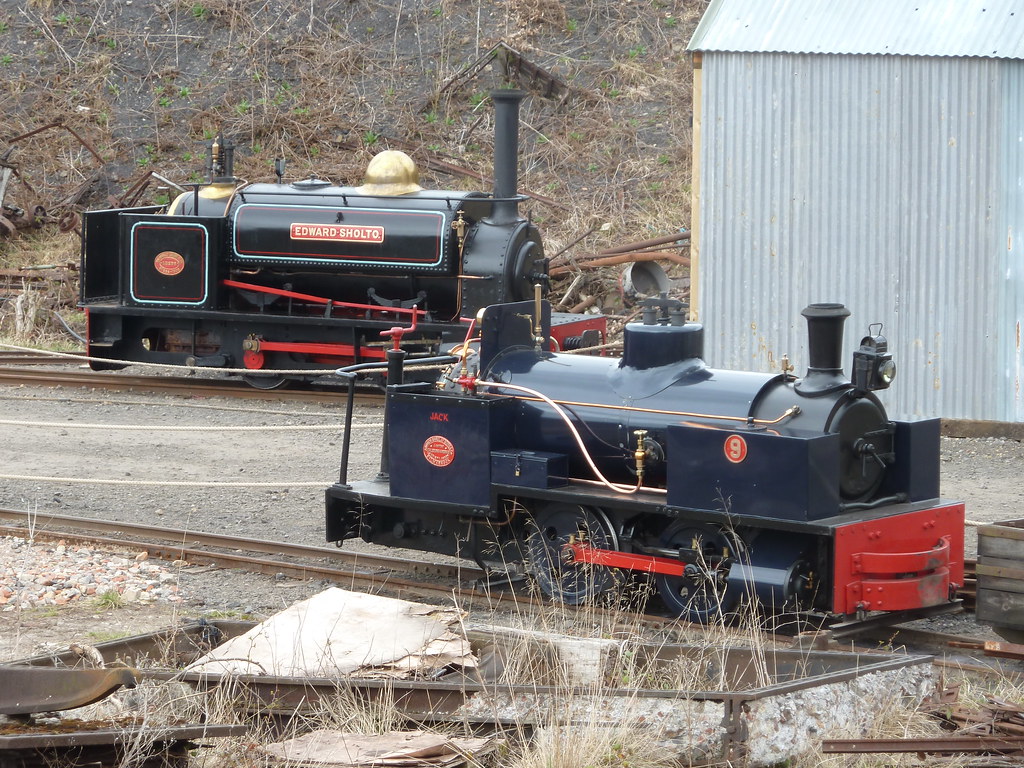This detailed image captures two vintage steam train engines positioned on separate tracks amidst a rocky terrain. The train in the foreground, slightly to the right, boasts a rich navy blue color with a striking red front bumper, red connecting rails, and a prominent gold-trimmed number 9 on its side framed by a red background. This engine also features intricate gold piping and a distinctive light on the front. Directly behind this train, on a parallel track, stands another striking steam engine, predominantly black with elegant gold detailing. The black train bears the name "Edward Sholto" in gold letters against a red background, and a red circular emblem towards its rear. Both trains are isolated, without any attached cars. The scene is complemented by a tin shed to the right of the blue train and a rugged hill adorned with sticks and rocks in the background. The area around the tracks features scattered gravel and additional rails, adding to the historic and rustic ambiance of the setting.